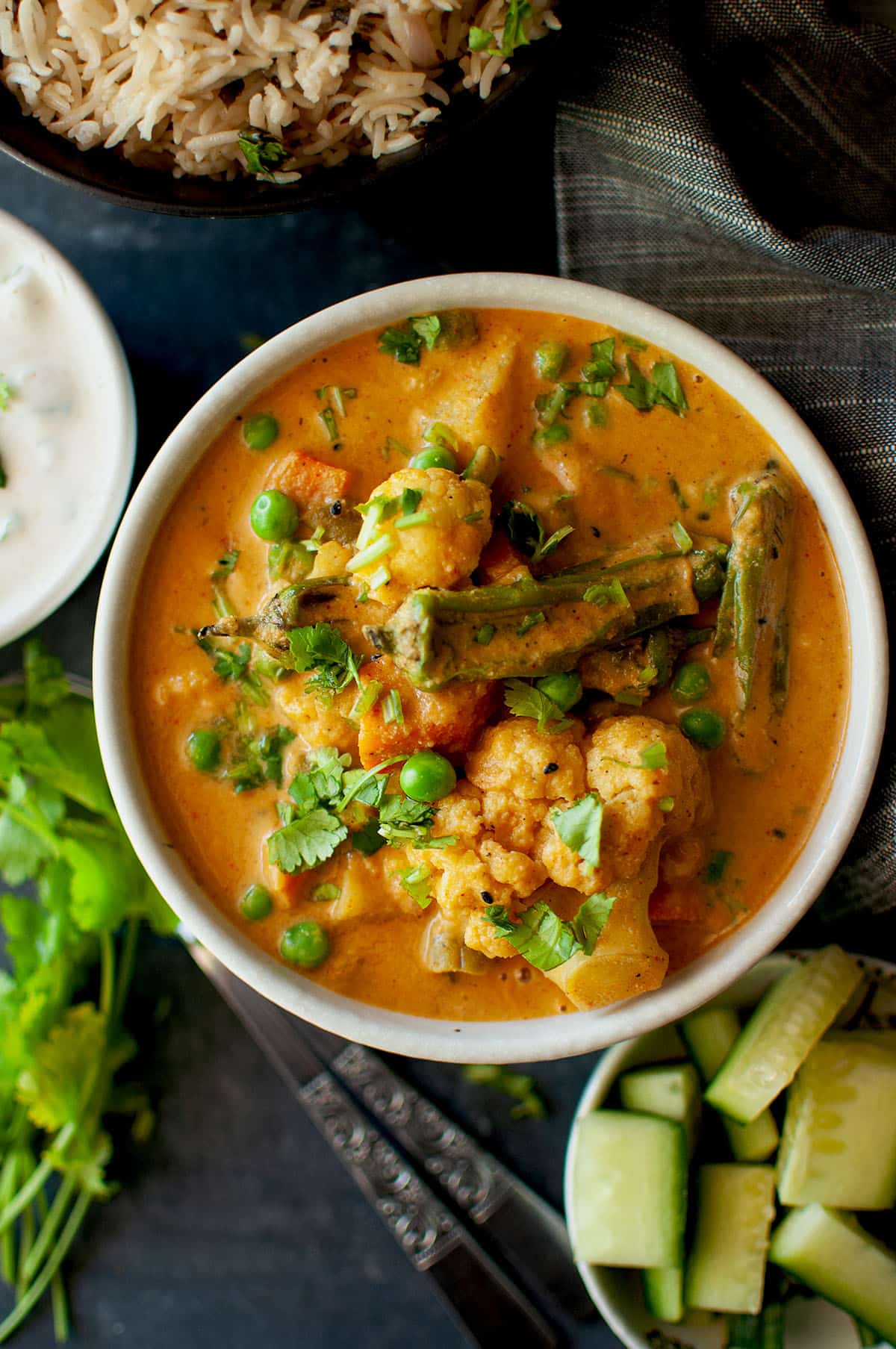In the center of the image, there's a white round bowl filled with a thick, orange viscous liquid, which appears to be a soup or stew. Inside the bowl, there are green peas, green stalks that could be celery or green beans, white bulbous pieces resembling cauliflower soaked in the vibrant sauce, and what look like croutons. The setup is on a dark-colored table or tablecloth, creating a stark contrast with the bright, colorful contents of the bowl. Scattered around the bowl are several other items: to the top left, a bowl of rice and below it, a bowl containing white sauce; to the bottom right, chopped cucumbers or squash; and flat herbs like cilantro are strewn across the table. Silver utensil handles, including a fork and a spoon, are visible at the bottom center. The top right shows glimpses of a tablecloth. The image gives a detailed and inviting presentation of a meal, with additional bowls containing food items blurred out in the background.